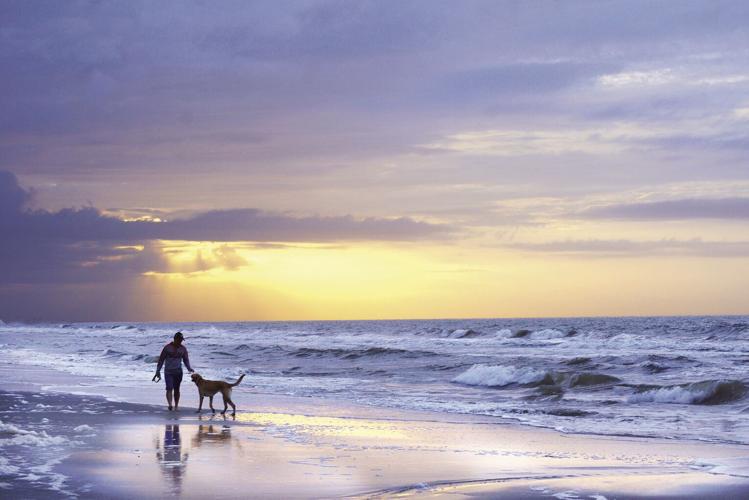This photograph captures a serene beach setting during an evening sunset. The sky, painted in hues of blue and silvery grey, is partly cloaked by clouds with a portion of the sun casting its yellow rays through them. The scene reflects beautifully on the glossy, wet sand, creating an iridescent effect that complements the deep blue and silvery waves lapping at the shoreline with visible white caps. In the foreground, a person in shorts and a hat walks along the damp sand with footprints trailing behind them, symbolizing their journey. They are extending a hand towards a tall, yellowish-brown dog that looks up at their owner attentively. Both the person and the dog are mirrored in the shimmering wet sand, adding to the tranquil ambiance of this picturesque moment by the ocean.